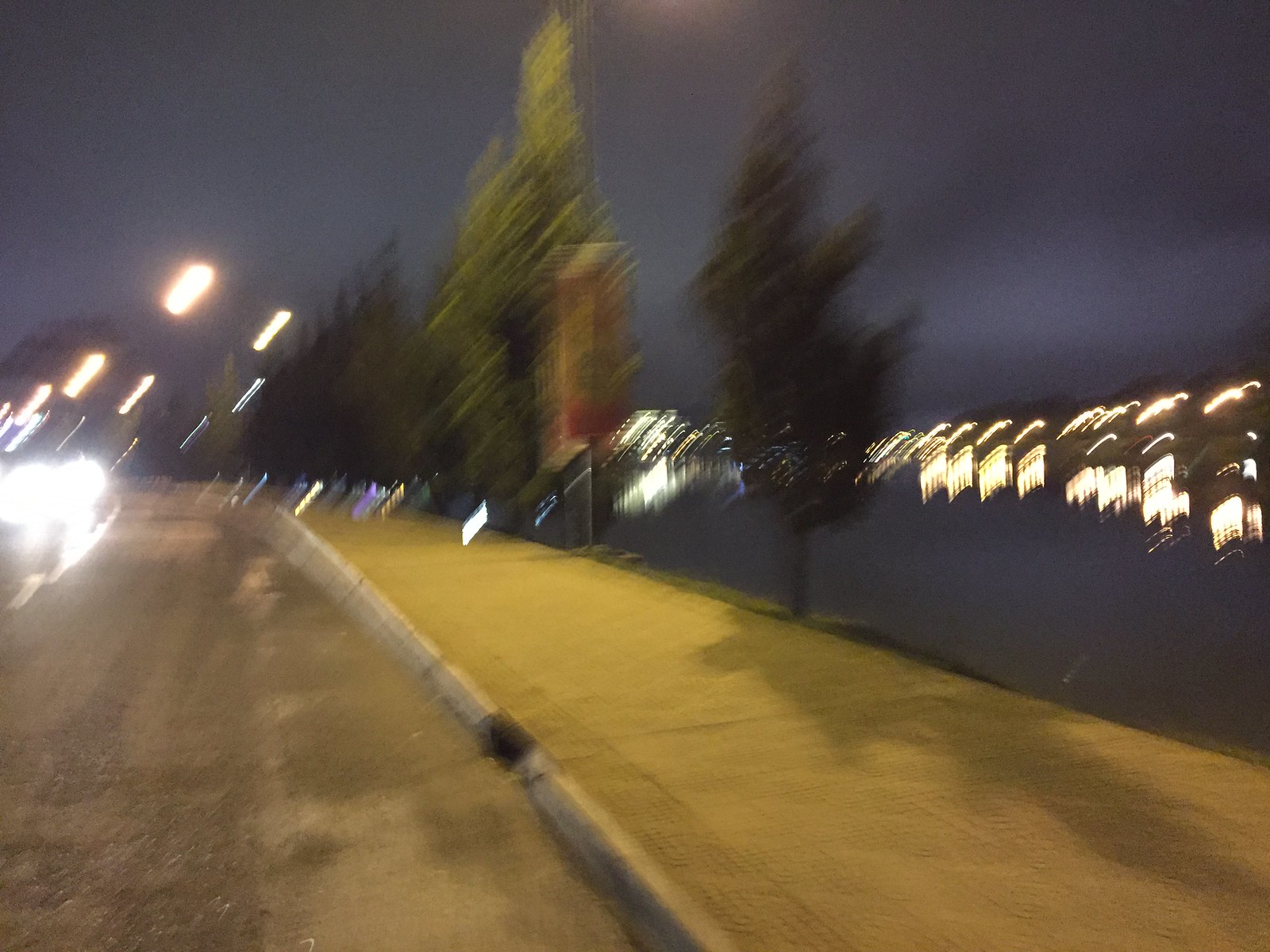A blurry nighttime photograph taken outdoors, likely at the edge of a waterway. The perspective seems to be from a roadside, capturing a gray asphalt surface with a light-colored curb. Adjacent to the curb is a light concrete sidewalk, bordered by several tall, thin trees. Beyond the sidewalk, a hill slopes down toward a dark grayish-blue reflective body of water, suggesting a nighttime overcast sky. In the background, there are blurred lights, possibly from houses, and bright oncoming traffic lights to the left, along with street lamps overhead, hinting at a busy area even at this late hour. The overall effect gives the impression that the camera was in motion, adding to the image’s blur.